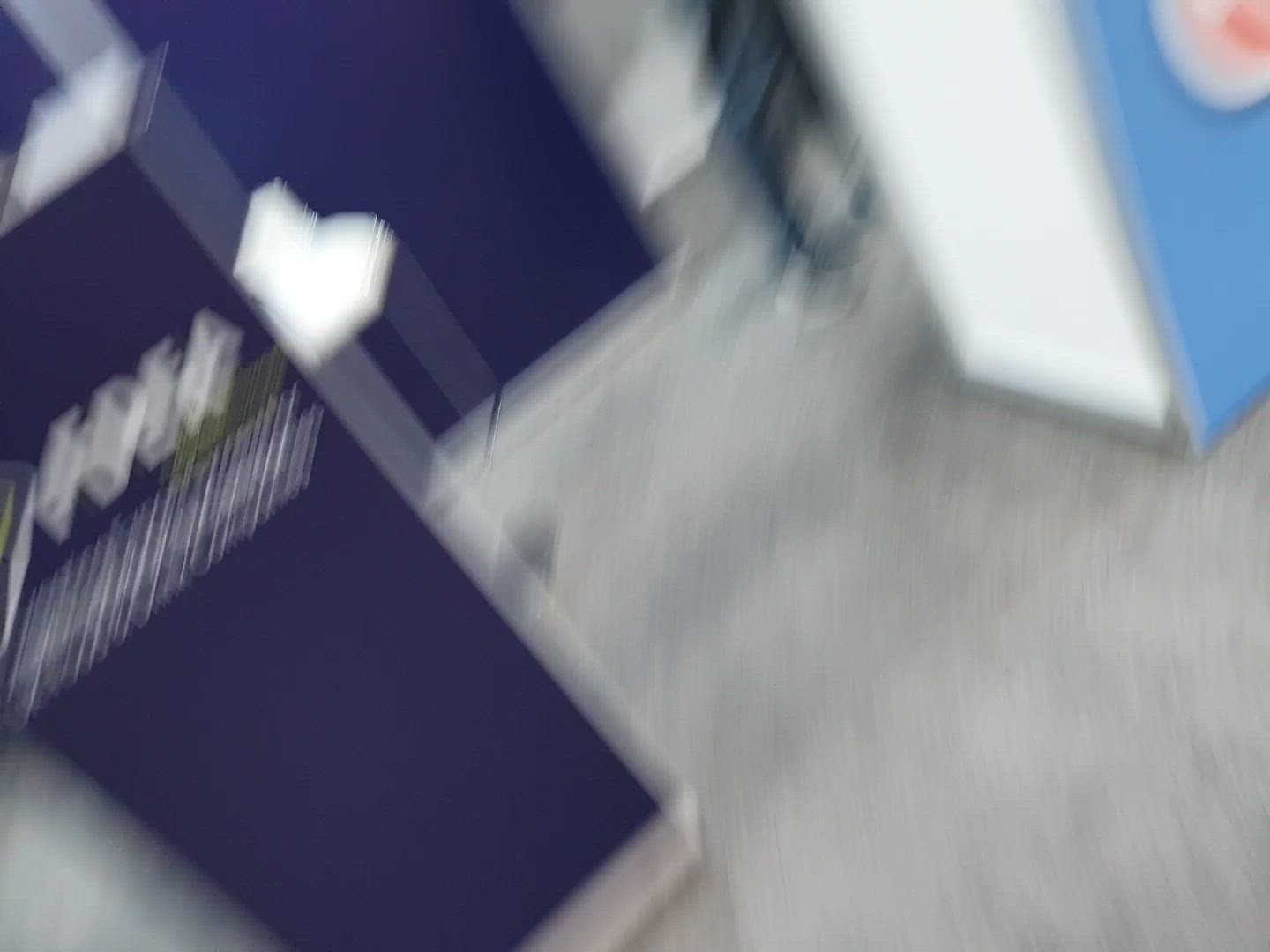This photograph, taken indoors, is very blurry, likely due to motion. The image showcases a scene within a building, characterized by a gray carpeted floor. In the background, multiple navy blue panels with indistinct white writing are visible against gray and white walls. One particularly noticeable navy blue panel features a circle with red coloring in the middle. To the right, a white wall can be seen, and beside it is a white and blue podium. The lower half of a person wearing tight denim jeans and gray tennis shoes with white laces is also visible. The photo includes additional elements like short streaks of color, possibly illustrating the movement. This well-lit interior, likely illuminated by standard office lighting, displays a mixture of various blue panels, gray carpeting, and some indistinct dark-colored objects, possibly furniture or decor, hinting at a structured, formal environment.